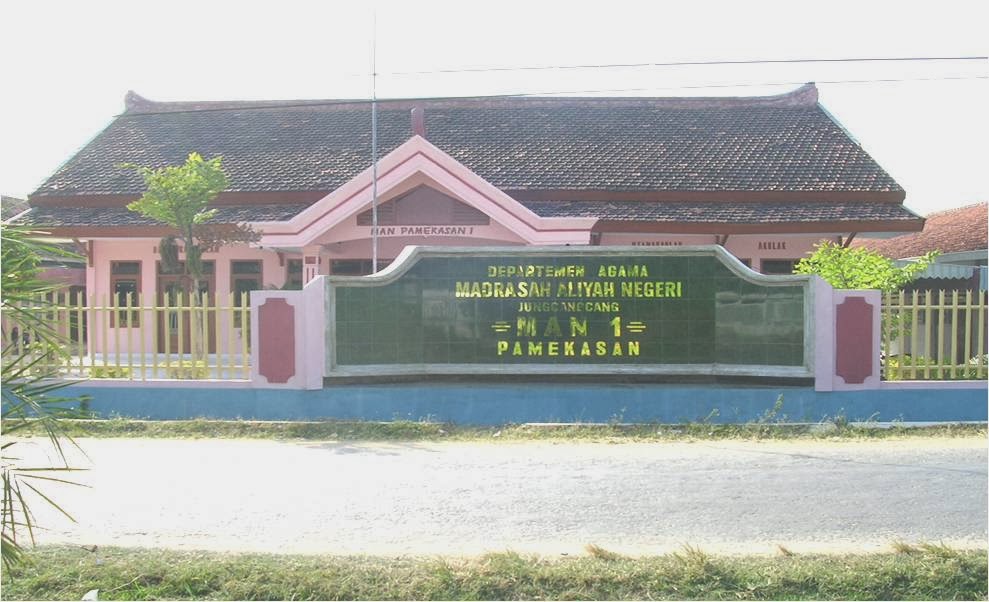The horizontal rectangular image captures an outdoor setting with a notable building situated behind a road that appears to be unpaved, possibly a dirt road. Dominating the foreground is a distinctive yellow fence featuring a blue bottom section. Centered in front of this fence is a large black tiled sign with pink edges and intricate designs, topped with gold lettering in a foreign language. The sign includes phrases such as "Department of Ghana" and "Man 1 Tamakazan." Behind the fence stands a pink-hued building with brick construction, adorned with oriental accents on its dark-colored, tile roof reminiscent of Chinese architectural styles. The entrance of the building is marked by a triangular arch and a foreign inscription that reads "Heng Peng Risen 1." The overall scene is framed by the contrast between the earthy tones of the road, the vivid colors of the fence, and the culturally distinct design elements of the building.